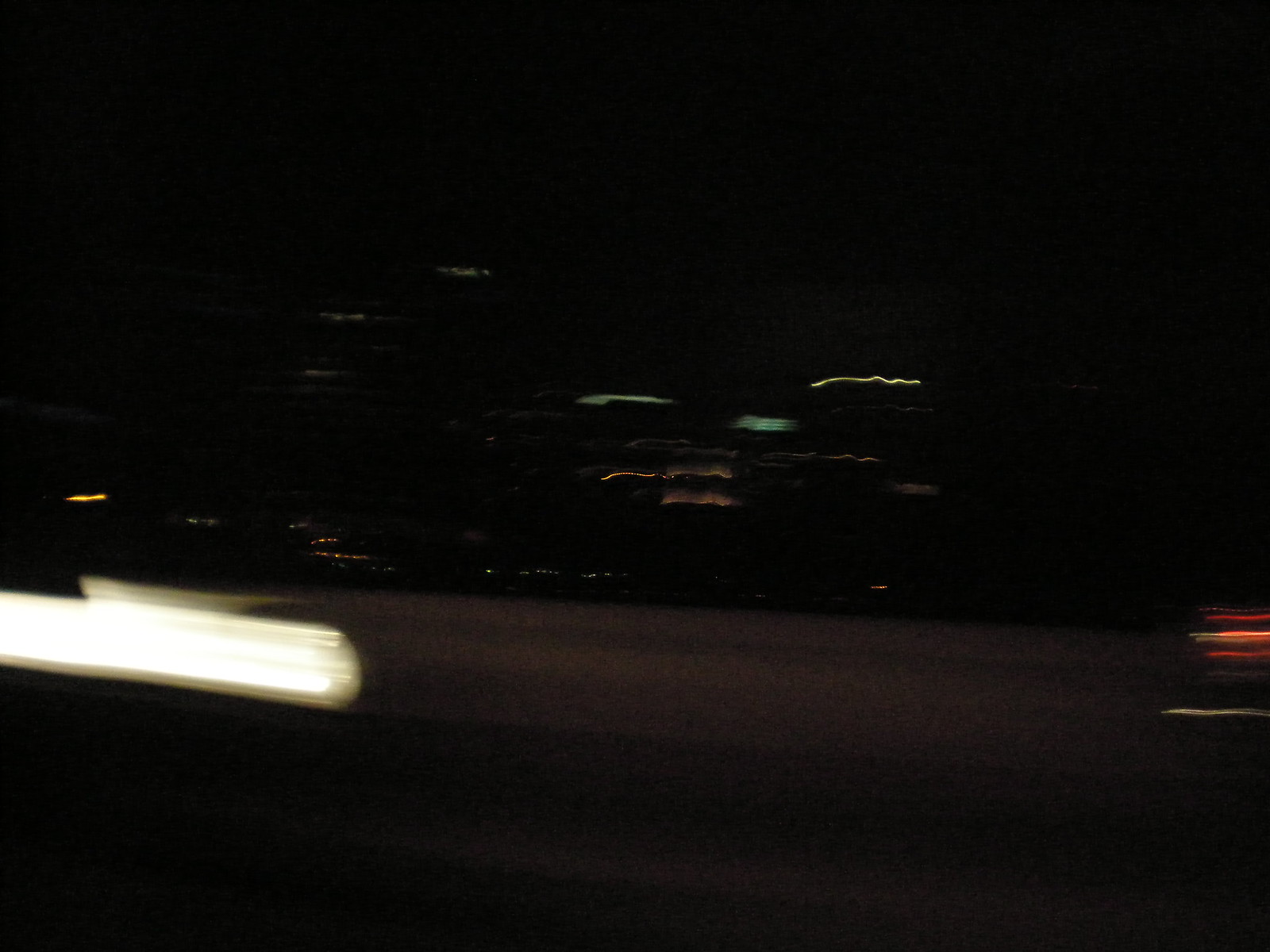A nocturnal, motion-blurred photograph captures the dynamic scene of what appears to be a car driving along a road. The right-hand side of the image is dominated by a vibrant streak of red light, likely the taillights of the vehicle, while the left side showcases a contrasting streak of white light, probably the headlights. Between these luminous trails lies a gray expanse, presumably the road. The overall picture is a dramatic smear of whitish-yellow, red, gray, and black hues, conveying a sense of movement and speed. The background is shrouded in darkness, punctuated by diffused spots of yellow and green light from a distant, illuminated area. Despite its blurriness, the photograph effectively captures the essence of nighttime motion.